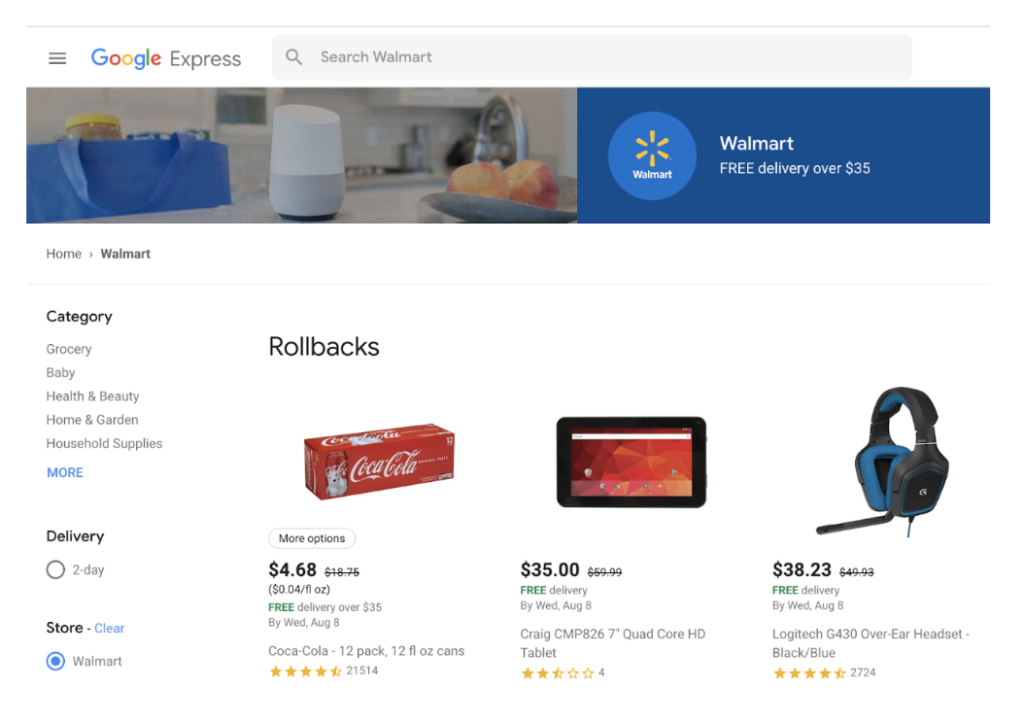The image displays a webpage with a clean and organized interface. At the top, there are three horizontal gray bars of equal size, stacked vertically, which likely serve as a menu icon. Next to it, the Google logo is prominently featured, followed by the word "Express." Below this, a gray rectangular search box with a magnifying glass icon is labeled "Search Walmart."

Occupying the upper midsection of the page is a banner. The left half of the banner showcases a blue bag filled with various groceries, including a visible jar of peanut butter, set against a white kitchen backdrop. In the kitchen, a Google device is placed on the counter beside a bowl containing peaches. The background also reveals a faucet and several containers on the back counter.

The right half of the banner contrasts with a dark blue background featuring a circle with a lighter blue interior. Inside the circle is the Walmart logo, accompanied by the text "Walmart" in white. To the right, additional text reads "Walmart, free delivery, over $45."

Below the banner, a vertical sidebar lists categories in a streamlined column. It starts with "Home" followed by arrows indicating nested options. Categories include "Grocery," "Baby," "Health and Beauty," "Home and Garden," "Household Supplies," and "MORE" highlighted in blue uppercase letters. Further options mentioned are "Delivery," marked with an open circle, "Two-Day," "Store," with "Clear" in blue, and "Walmart" also in blue, which appears to be the selected option. 

"Rollbacks" is another section listed with three featured items, one of which is a 12-pack of Coca-Cola. This comprehensive layout aims to simplify navigation and enhance the user's shopping experience.